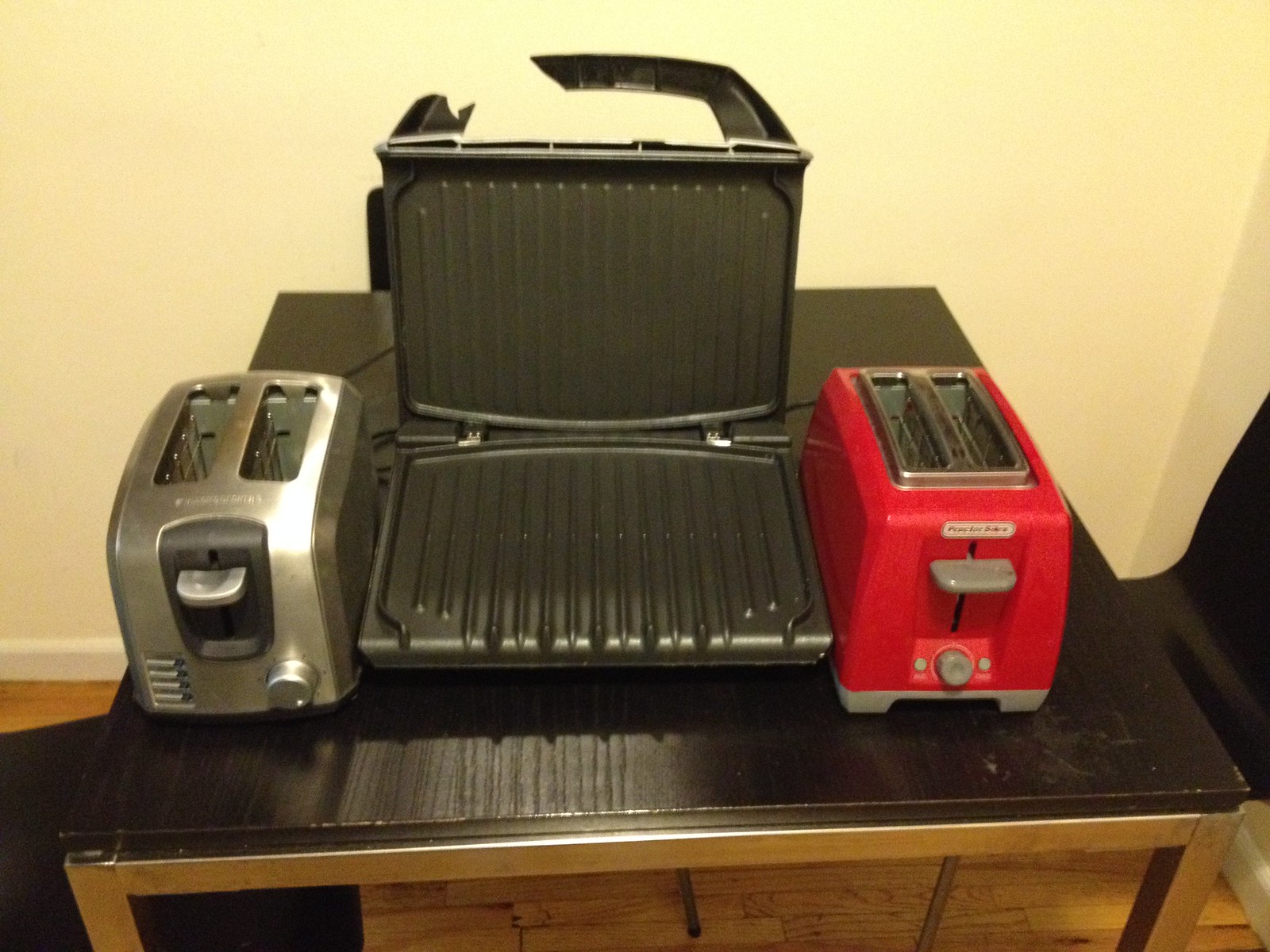In this interior photograph, a black table with silver metal legs is centered against a yellowish wall. On the table are three different toasting appliances. On the left side is a silver toaster with wide, rectangular slots and a lever and knob on the front. The toaster on the right is a red, boxier model with similarly wide slots and sleek silver and gray accents. Between these two toasters sits a larger, black sandwich grilling machine with a hinge, which is open, revealing grooved surfaces designed to grill both sides of a sandwich simultaneously. Additionally, there is a box of tissues visible behind the appliances. The scene is further framed by a white section of the wall on the left and an indistinct black object on the right, possibly a chair.